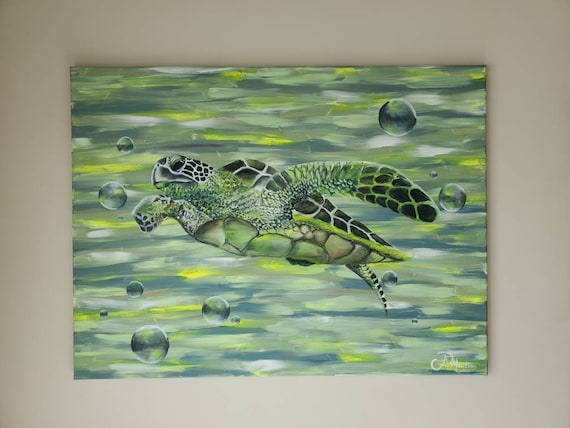The artwork is a detailed canvas painting depicting a green sea turtle swimming in water. This rectangular piece hangs on a white wall and showcases an abstract background composed of various shades of green, including light green, dark green, lime green, along with whites, yellows, and hints of blues and grays. The background is designed to evoke the appearance of waves, interspersed with bubbles of varying sizes, particularly noticeable in the bottom left and top right of the painting. The turtle, viewed from a side angle, features a scaled, plated look on its back, tail, head, and flippers. Its shell is slightly darker than the rest of its body, with intricate patterns. A white signature, though too small to read clearly, is visible in the lower right corner of the artwork.